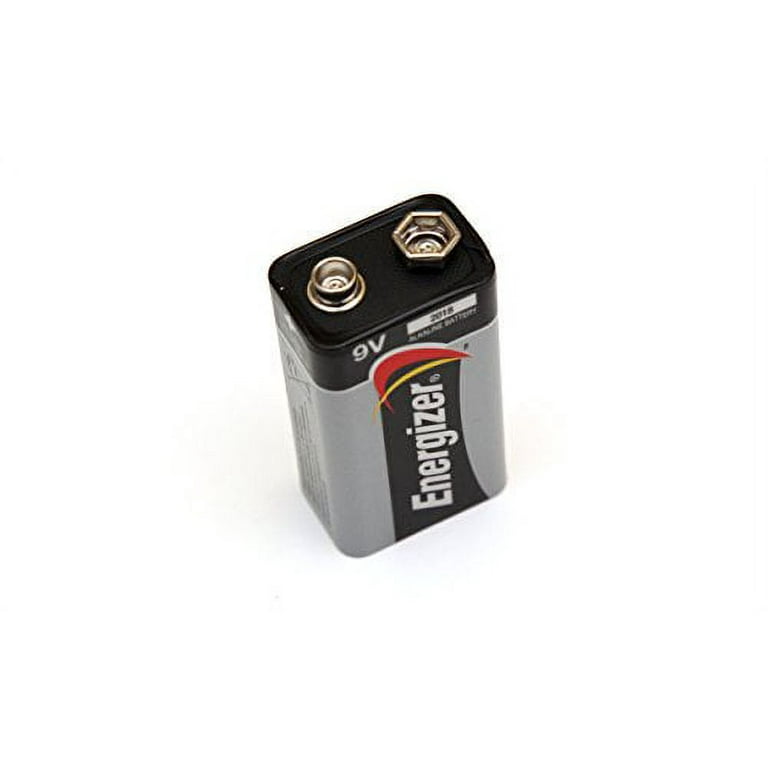The image showcases a 9-volt Energizer alkaline battery set against a white background, taken from an isometric view allowing visibility of both the front and top. The battery is rectangular with slightly rounded edges, featuring a gray body and a black top. Centered vertically on the front, a black bar displays the brand name "Energizer" in bold white letters. Above this, there's a red, boomerang-like logo with a thin yellow line below it. Prominently marked in white on the black top is "9V" signifying nine volts. Additionally, a white horizontal box with black "2018" text is located above the logo. Topside, there's a circular silver metal connector on the left and a hollow hexagonal silver connector on the right, denoting the battery's terminals.